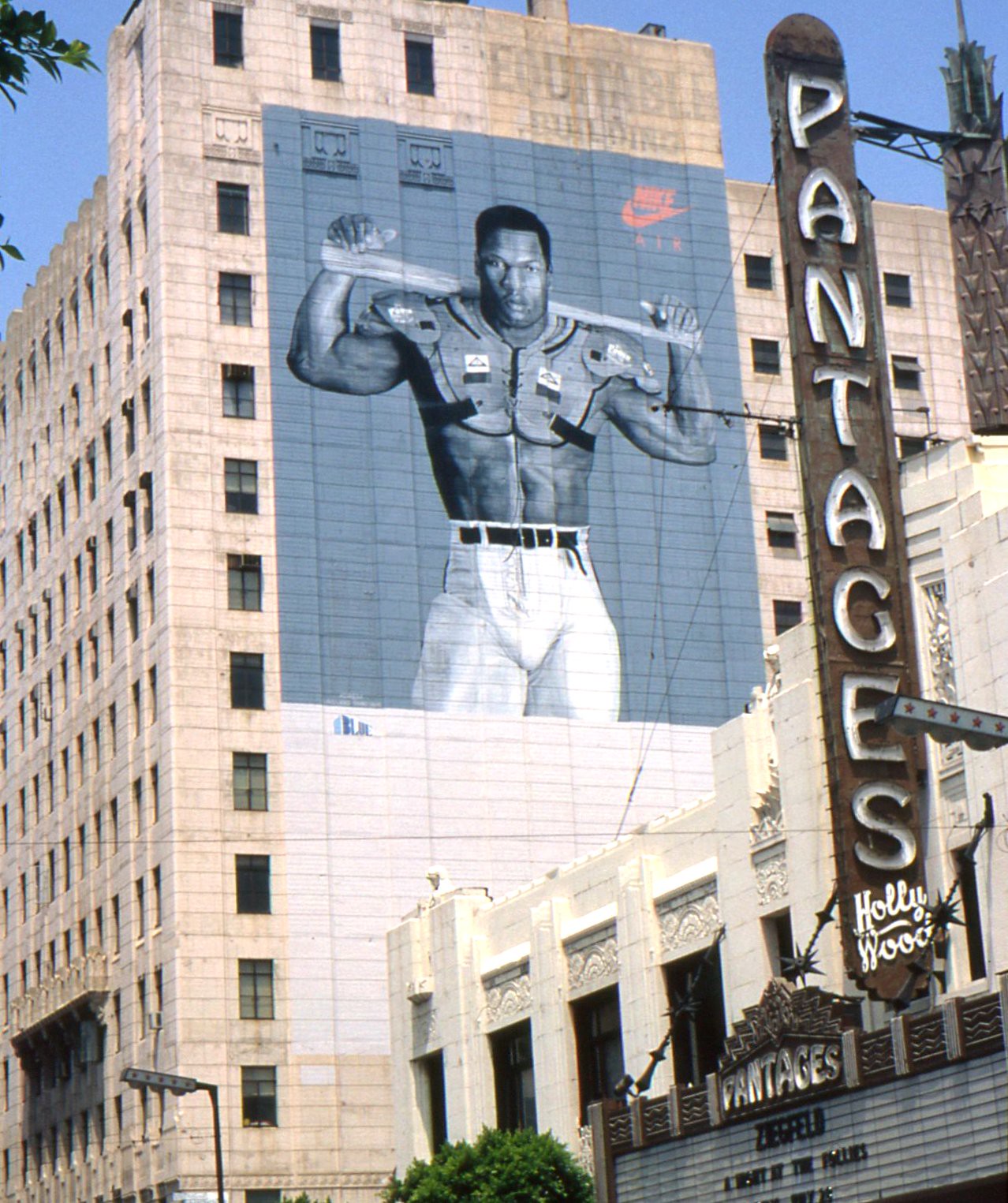The image showcases the side of a tall, 12-story beige stone building prominently featuring a massive, six-story-high Nike ad. The advertisement depicts a muscular African-American athlete, bare-chested with shoulder pads, dressed in belted white pants, and posed powerfully with a baseball bat resting behind his neck, held by both hands. The dark grey background of the ad contrasts sharply against the white stone of the building, emphasizing the athlete's strong presence. In the upper right corner of the ad, the iconic red Nike Air logo is clearly visible. Below this building, another structure with a marquee proudly displays "Pantages Hollywood," adding an element of urban sightseeing to the vibrant street scene.